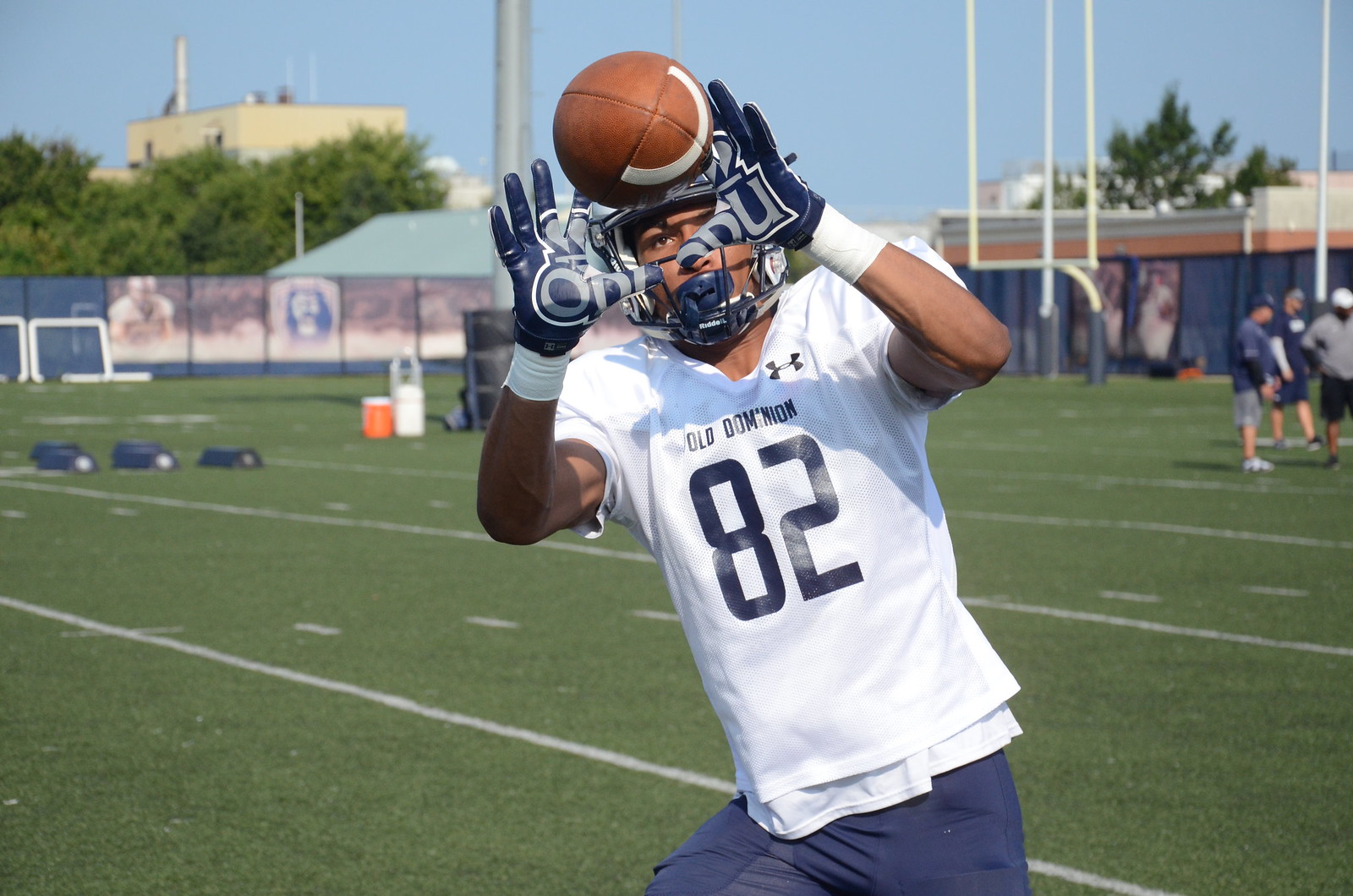In this action-packed image captured during daytime football practice, a player from Old Dominion, clad in a white jersey with the number 82 in navy blue and blue practice shorts, is poised to catch a brown football with a white stripe. His dark blue gloves and brown wristbands add extra support, and a blue mouth guard accompanies his protective helmet. The scene is set on a green football field marked with white lines and surrounded by a barricade, with a light yellow field goal post also visible. In the background, several coaches dressed in blue school-themed apparel, including short-sleeve shirts and shorts, observe the practice. An orange Gatorade container sits nearby, and beyond the field, there's a mix of trees, a factory-like building, and various indistinct signs on a fence. The sky above is a clear, vibrant blue, framing the dynamic moment of the player bracing to catch the oncoming football.